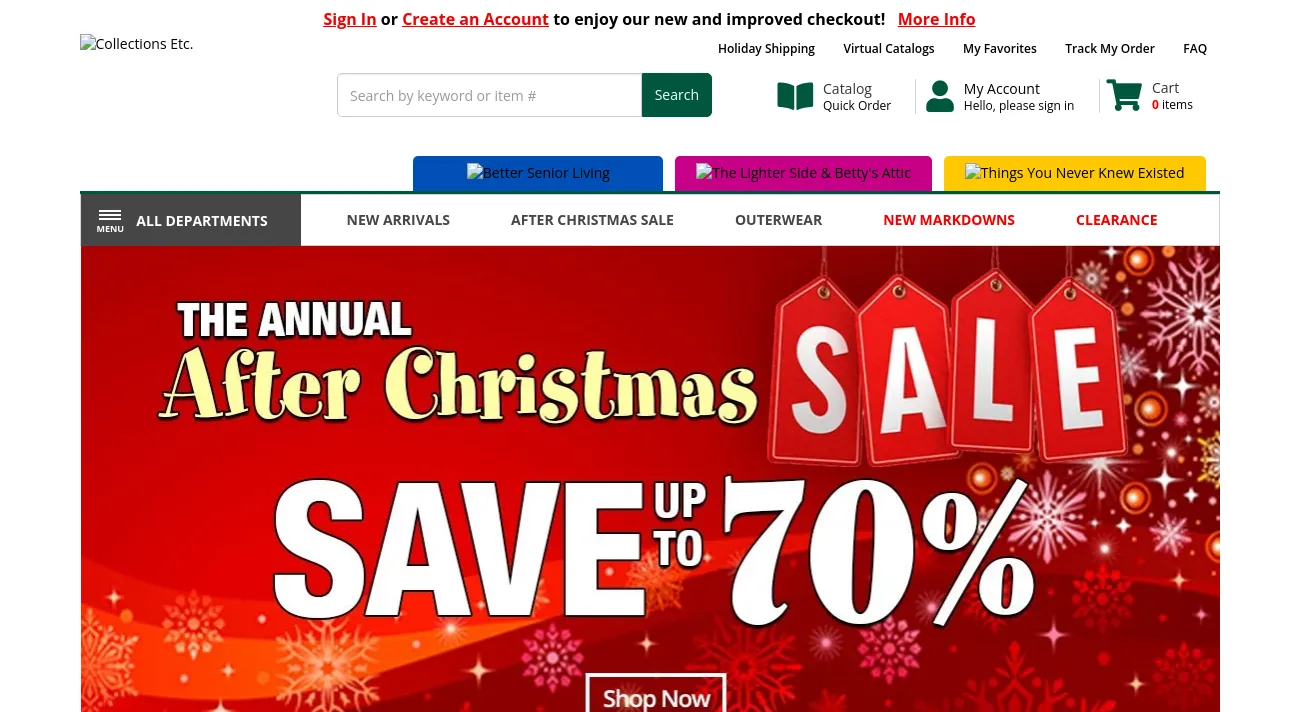The website interface is primarily set against a white background with black text. Centrally located is a prompt inviting users to "Sign in or create an account to enjoy our new and improved checkout," accompanied by a "More Information" link. The options for "Sign In," "Create an Account," and "More Information" are highlighted in red for emphasis.

Beneath this notice is a centered search bar with the placeholder text "Search by keyword or item number" in gray. The search bar is outlined in gray, and the search button on the right is green with the word "Search" in white.

On the right-hand side, there's a series of navigation links and account features, starting with "Holiday Shipping," "Virtual Cards," "My Favorites," "Track Order," and "FAQs." Lower down are additional options: "Catalog" and "Quick Order," represented with an icon of a book, followed by "My Account." This section includes the greeting, "Hello, please sign in," with a person icon, and a shopping cart icon in green showing "0 items."

Further down, the interface displays a row of tabs for different categories: "Better Senior Living" in blue, "Lighter Side" in pink, and "Betty's Attic: Things You Never Knew Existed" in yellow. These sections are followed by a horizontal navigation bar.

On the left side of the navigation bar, there is a gray button with three stacked lines, indicating a menu for 'All Departments.' The background from this point is white with black text, listing categories such as "New Arrivals," "After Christmas Sale," "Outerwear," and "New Markdowns" and "Clearance," both highlighted in red.